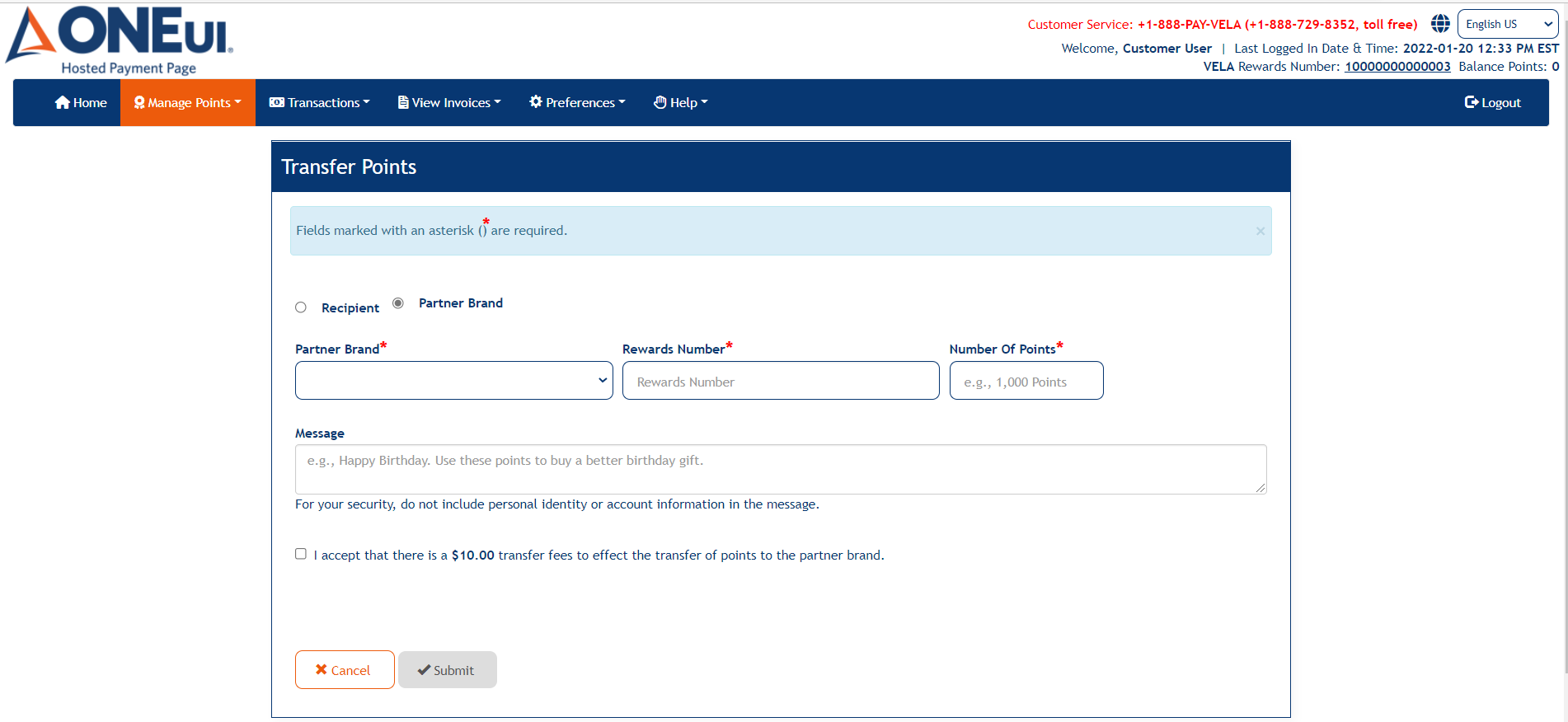The website displays the interface for 1UI, prominently featuring their logo — a combination of "1UI" in blue font accompanied by a blue and orange triangle. In the top-right corner, there's red font text, too small to decipher, followed by two lines of navy blue text and a drop-down box labeled "English US."

Directly beneath this header is a blue navigation bar with menu options in white font: "Home," "Manage [unreadable]," "Transactions," "Out View," "Invoices," and "Help." The second menu option is highlighted in orange, indicating the current section. On the far right of this menu bar is a logout link.

Further down, a blue banner states "Transfer Points" in white font. Below it, there's a light blue rectangular box containing small, unreadable text. The main section of the page has a white background with blue font, featuring several radio buttons and three input fields, followed by a message field.

At the bottom-left of this section, there are two buttons: a white "Cancel" button with red font and a gray "Submit" button with blue font.